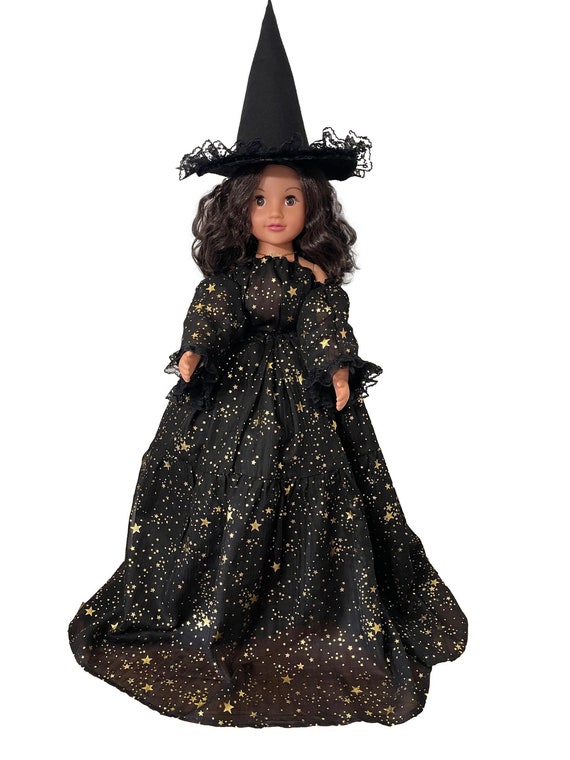The image depicts a charming witch doll designed to resemble a child. The doll has a peach-toned complexion and features big brown eyes, red-pink lips, and long, flowing brown hair that cascades down to her shoulders. She is dressed in a black witch's dress adorned with gold stars, creating an enchanting celestial pattern reminiscent of a starry night sky or a golden galaxy. The dress reaches the bottom of the image, touching a white background but not the doll itself. Her hands extend out in front of her, and she wears a prominent, black witch's hat with frills around the brim. The hat sits tall on her head, directly above her forehead. The doll's expression is friendly, with a smile visible on her face, and she wears a small necklace as an accessory. The overall setting of the photo focuses solely on the doll, emphasizing her detailed costume and endearing appearance.